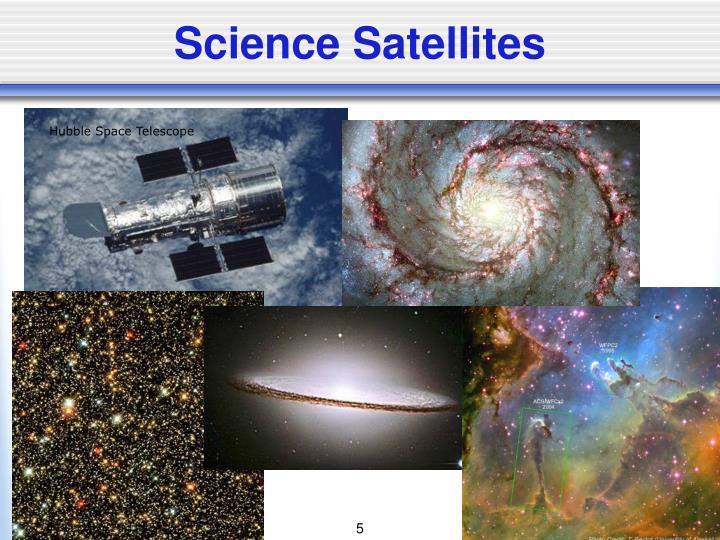This image, titled "Science Satellites," features a collage of five distinct space-related photographs arranged over a white background. The top portion of the image has a gray-striped border with a blue line at the bottom and the title "Science Satellites" in blue font. The upper left corner displays a photograph of the Hubble Space Telescope, characterized by its shiny metal, foil-like surface, and four solar panels, floating above the Earth’s blue surface and white clouds. The telescope appears to be a composition of two cylindrical structures, with the front shield open. Adjacent to this on the top right is a glowing, reddish-brown swirling nebula. On the bottom left, a constellation of bright stars set against a black background represents the vast cosmos. The center-bottom image likely illustrates a solar system. Finally, the bottom right depicts another intricate nebula, capturing the awe-inspiring complexity of stellar nurseries. A small number 5 is inscribed at the very bottom of the image, indicating its possible sequence in a series from an educational or scientific website.